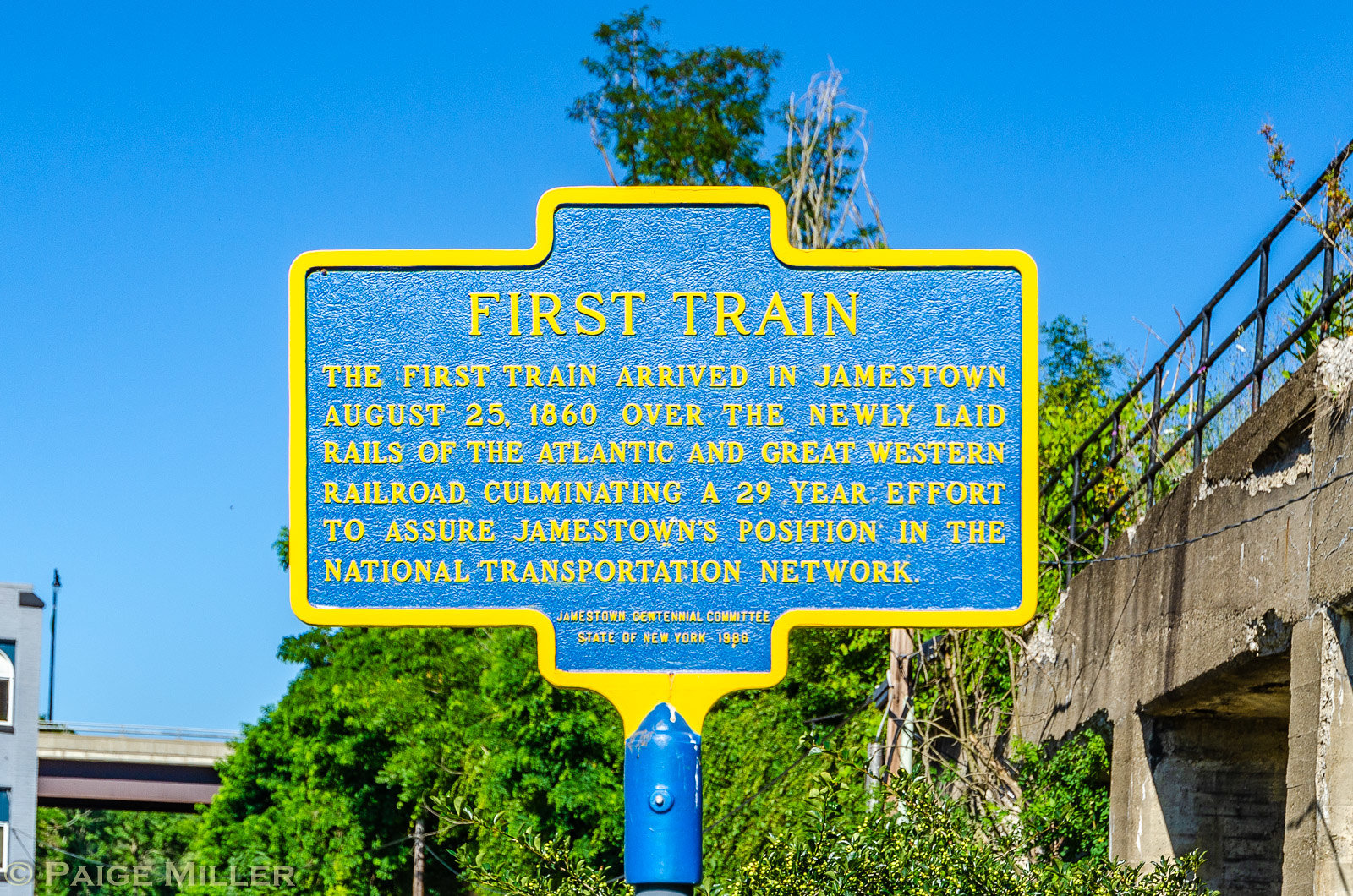This is a horizontal rectangular photograph taken outdoors during the daytime, capturing a historical marker against a backdrop of vibrant blue sky that lightens towards the lower left corner. Dominating the upper portion of the image is a large green tree, and next to it, partially visible, is an old viaduct with crumbling concrete and a black railing on the right-hand side. The central subject of the photo is the historical marker, which is mounted on a blue metal post. The marker itself is also blue with a gold outline and gold-raised lettering. At the top, the inscription reads "First Train." Below, it continues: "The first train arrived in Jamestown August 25th, 1860, over the newly laid rails of the Atlantic and Great Western Railroad, culminating a 29-year effort to assure Jamestown's position in the National Transportation Network." Beneath this text, in smaller, less legible gold letters, it reads: "Jamestown Centennial Committee, State of New York, 1986." This detailed scene captures both the historical significance and the serenity of the location.